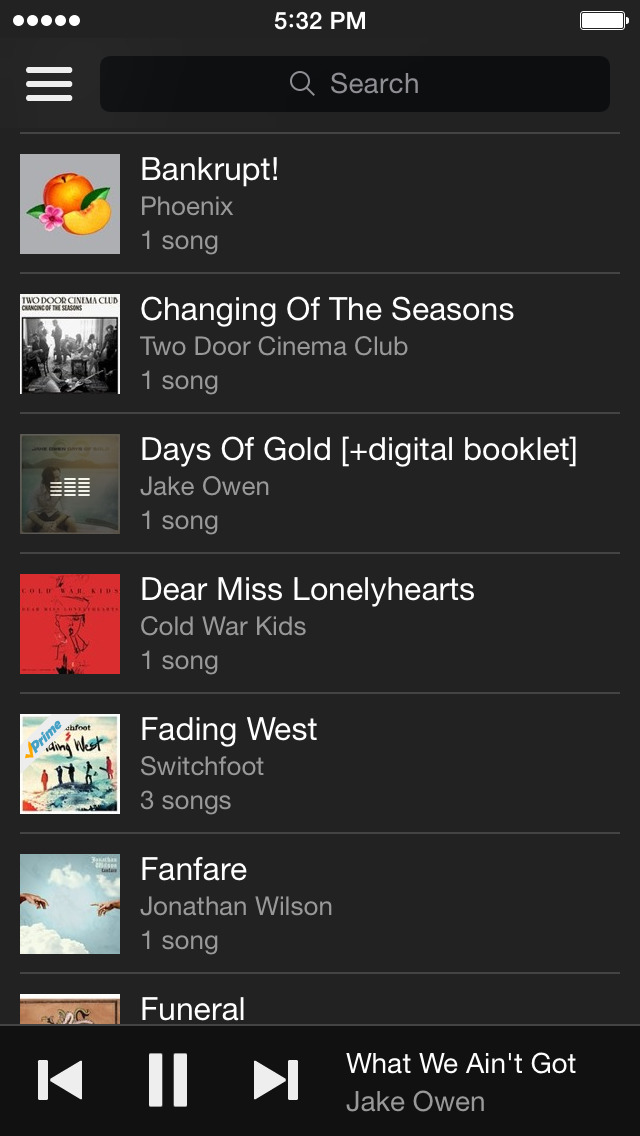The image displays a music streaming interface, likely from a mobile device or a widget. The top center of the screen shows the time as 5:30 PM, while a full battery indicator is located at the top right corner. There are no visible Wi-Fi or cellular signal indicators. The overall color scheme is primarily black with varying shades, while most of the text is in white, except for the grey search bar at the top featuring the word "Search" and a magnifying glass icon.

Beneath the search bar, there are seven thumbnails, each representing different songs or albums. The visible titles include "Bankrupt," "Changing of the Seasons," "Days of Gold" (noted as a digital booklet), "Dear Miss Lonely Hearts," "Fading West," "Fanfare," and "Funeral." At the very bottom of the screen are playback controls, including previous, pause, and forward buttons. The currently playing song is "What We Ain't Got" by Jack Owen.